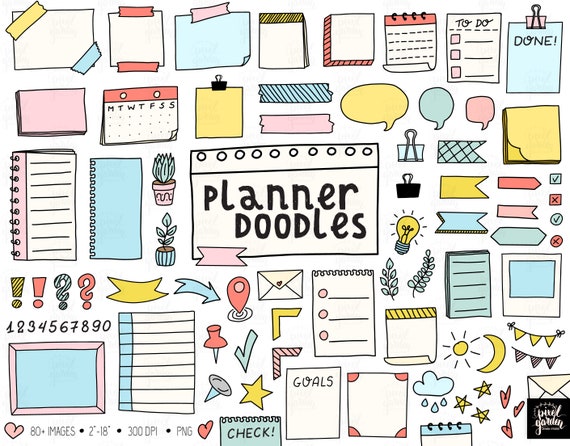The image contains whimsical illustrations of various notebooks and office supplies, arranged in a colorful, eclectic manner. The center features a white text box styled as a notebook, complete with hole punches and pink tape at the top, boldly displaying the words "Planner Doodles" in black text. Surrounding this central element are numerous depictions of stationery items: calendars, phone books, whiteboards, lined papers labeled with tasks like "goals," "check," and "done," and various sticky notes in different colors pinned with colorful tapes and clips. Additionally, the image includes elements like paper clips, light bulbs, thumbtacks, a to-do list, and small houseplants interspersed with playful doodles of rain clouds, suns, moons, stars, banners, envelopes, speech bubbles, numbers, and location icons. A note at the bottom left mentions the inclusion of 80 images ranging in size from 2 to 18 inches at 300 dpi in PNG format. In the bottom right corner, an unreadable logo is present.